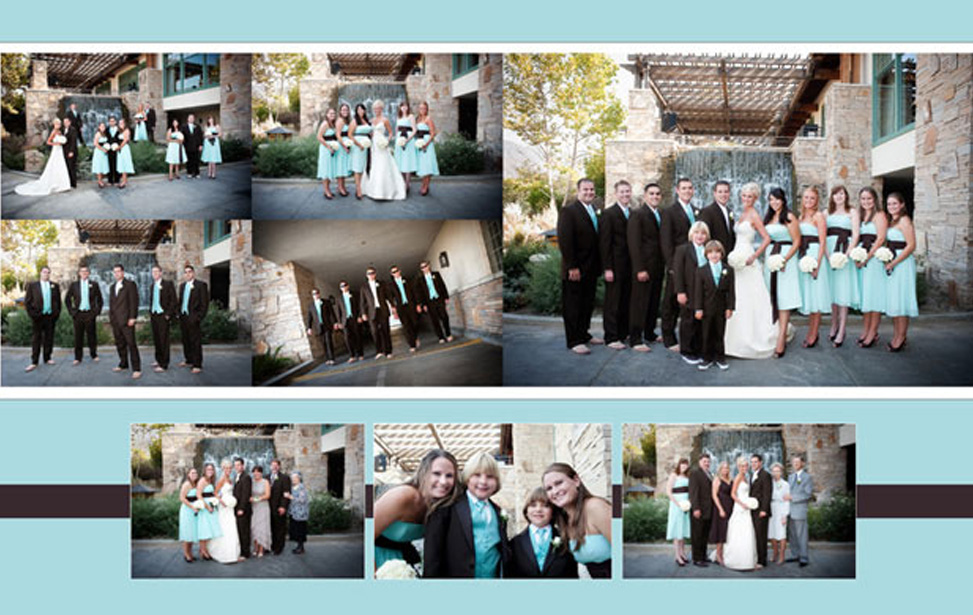The image is a rectangular wedding collage approximately five to six inches wide and four inches high, divided into two main sections. The top half of the collage is bordered by thin light blue and white lines and consists of five images. On the left side, there are four smaller images in a 2x2 grid. The upper left image features the bride and groom, while the upper right showcases the bride with her five bridesmaids dressed in light sea-green dresses with black belts. The bottom two images capture groups of groomsmen in dark suits. To the right of these four photos, a larger image shows the entire bridal party posed together; the groom and groomsmen in dark suits and the bride standing in her white wedding dress.

The lower half of the collage provides a blue background with a brown pinstripe running horizontally across the center. It contains three smaller photos. From left to right, they depict the bride and groom with family and children, including the ring bearers. Each image aligns with the same light sea-green and brown color scheme present in the bridesmaids' dresses and other elements of the collage.

This detailed and harmonious arrangement of images beautifully captures the essence of the wedding, showcasing the happy couple, their bridal party, and family members, all framed within a consistent and elegant color theme.